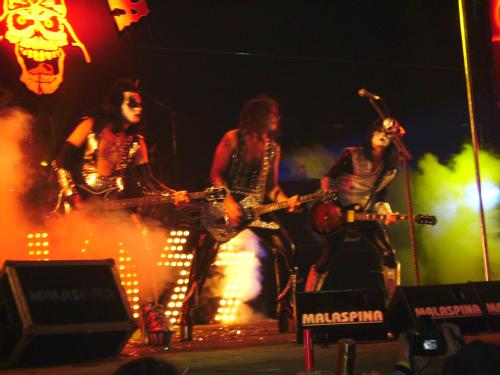This is a nighttime photograph capturing the iconic band KISS during a concert. Bathed in stage fog and clad in their signature black leather outfits with black and white face makeup, three guitarists, likely including Gene Simmons and Ace Frehley, energetically perform at the front of the stage. Behind them, the brightly lit "KISS" logo illuminates the scene. Hovering above in the upper left corner, a menacing, smiling skull with a helmet adds to the theatrical ambience of the show. Prominently placed at the lower left are large speakers facing the audience, each adorned with the word "Malaspina." The image, slightly blurry, indicates it might be an amateur shot from the late 70s, capturing the raw and electrifying atmosphere of a KISS concert.